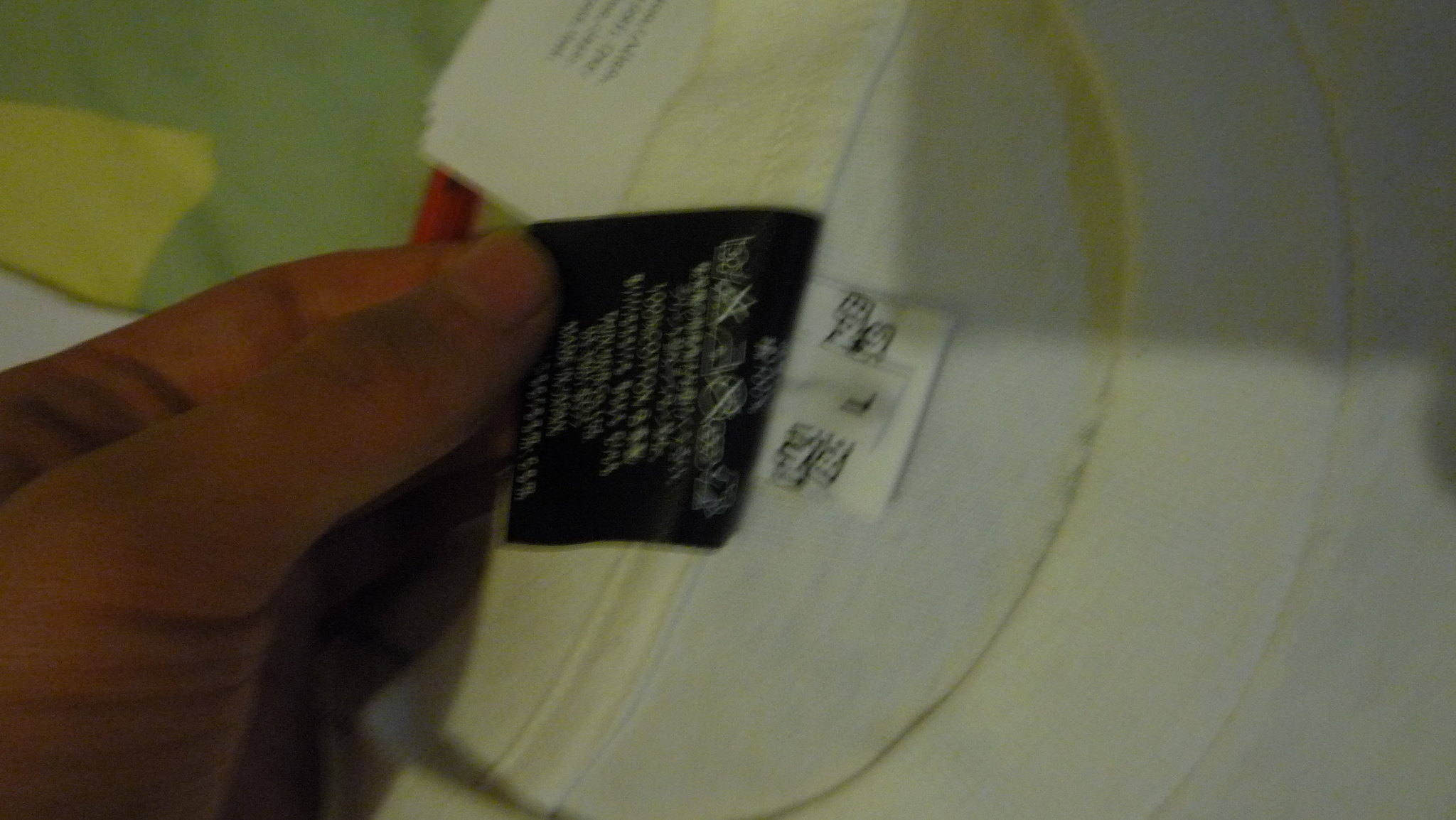In this photograph, a pair of hands holds up the top labels of a white shirt, which appears slightly yellowed and is shown from a fairly zoomed-in perspective. Due to the proximity and angle, much of the shirt itself is not visible, though the collar suggests it is a shirt. The image is somewhat blurry and dark, with noticeable shadows adding to the overall dimness. The primary label being held up shows the backside, rendering its text reversed and illegible, though the distinct outline of washing instructions is discernible. Below this label, another tag indicates the shirt's size as large ("L"), and beneath that, a partially obscured brand label is just visible but unreadable.